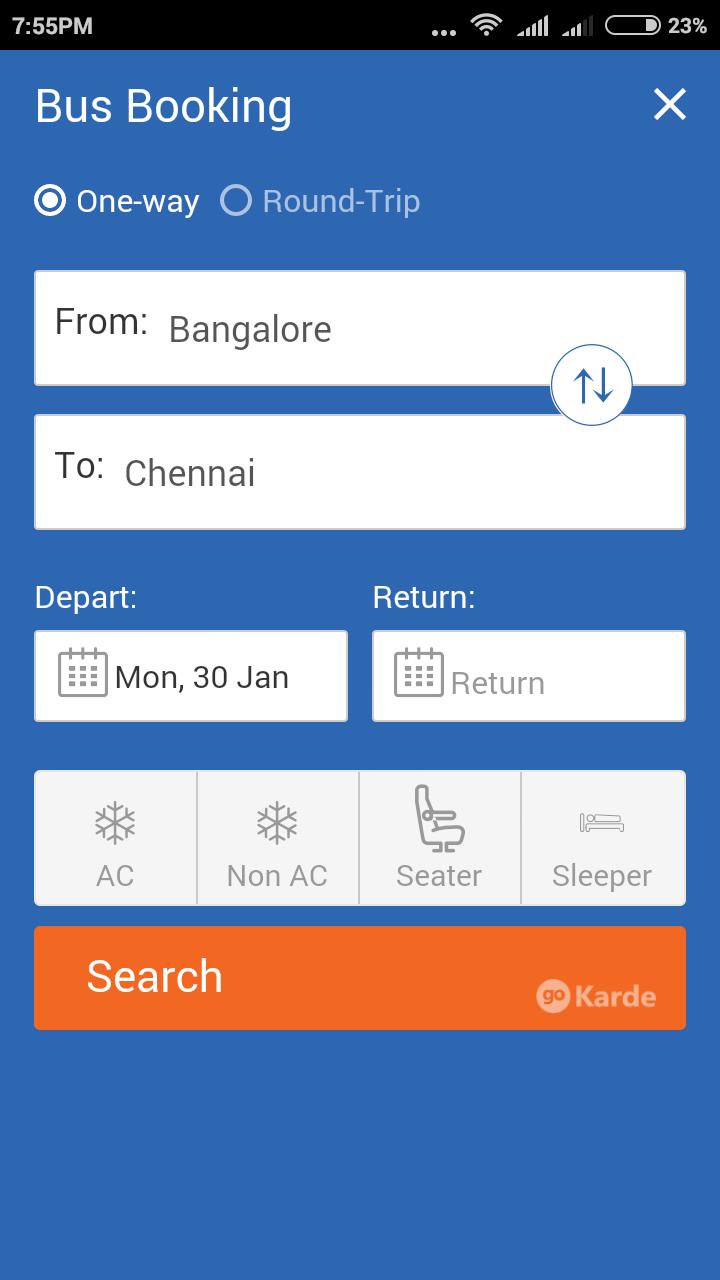This image is a screenshot taken from a smartphone displaying a bus booking website interface. The very top border of the screen is black, featuring the current time "7:55 PM" in white font on the left side. On the right side, a battery icon indicates a 23% charge, accompanied by two wireless connection icons and a Wi-Fi symbol.

The website's background color is blue, and in the upper left corner, the text "Bus Booking" is visible in white font. On the upper right corner, there is a white 'X' icon for closing the screen.

The user has selected a one-way trip option; the alternative would have been a round trip. Below this option, there are two white rectangles: one showing the departure city "Bangalore" and the other showing the destination city "Chennai."

Under these rectangles, there are two additional ones for selecting travel dates. The departure date is set to Monday, January 30.

Further down, there are four white rectangles divided into sections labeled "AC," "Non-AC," "Seater," and "Sleeper" in light grey font, representing different bus types. Below these options is an orange rectangle that functions as the search button, displaying the word "Search" in white font on the left side.

At the bottom of the screen, the company name "Karde" appears in white font, with a white circle next to the letter 'K' and the word "go" written in orange font.